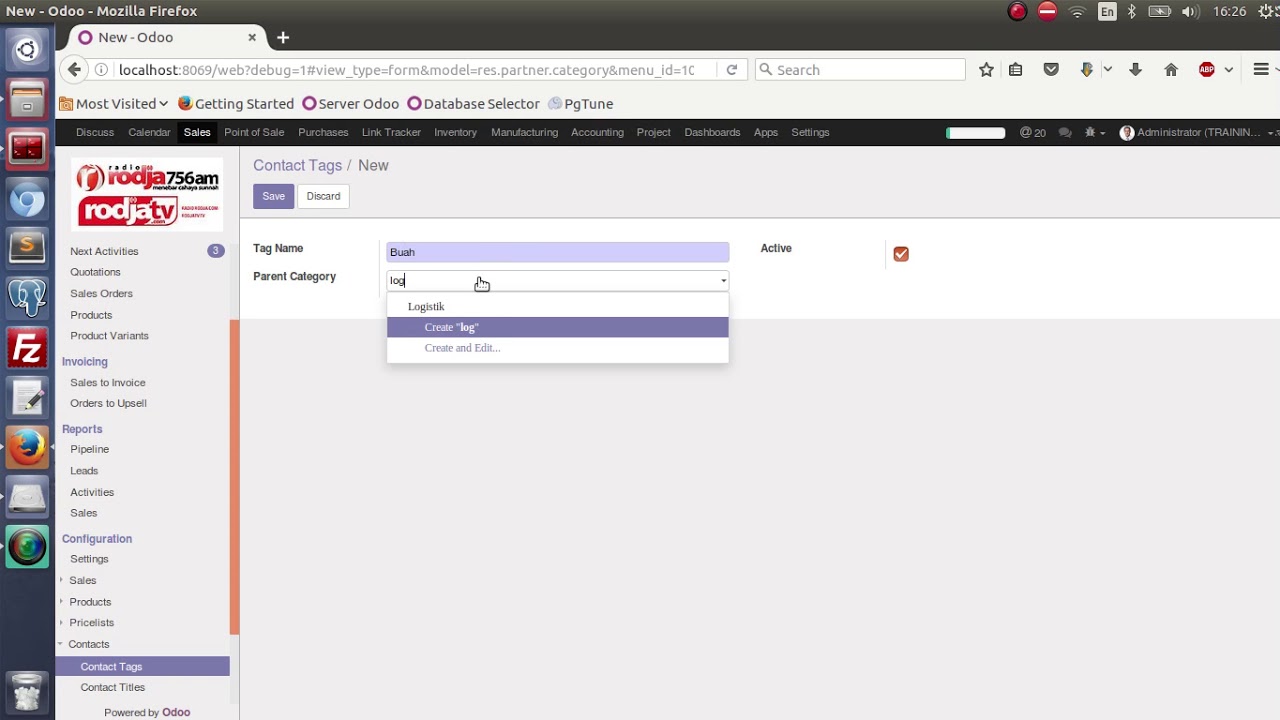This image showcases a newly launched website displayed on the Mozilla Firefox browser, specifically under the URL "localhost" indicating it might be a locally hosted development site for Odoo. 

On the far left of the screen, there's a black vertical navigation bar featuring various icons representing companies, such as one labeled "FZ." Notably, there is also a blue-colored Google Chrome icon and an icon depicting a world, which is green. 

The main section of the webpage prominently displays text reading "RODEO 756 AM." Along the left-hand side, a list of categories is visible, including "New," "Next Activities," "Quotations," "Podcasts," "Introducing Assist Salem to Invoice," "Orders," and others that are difficult to discern. Additional categories include "Reports" and "Configuration."

In the central body of the webpage, there are sections labeled "Save" and "Discard." There are fields tagged with names such as "Bush," and "Parent Company," accompanied by another text field marked "Log." A dropdown menu labeled "Log HIC" is also present. The page indicates an active status with a red square containing a check mark.